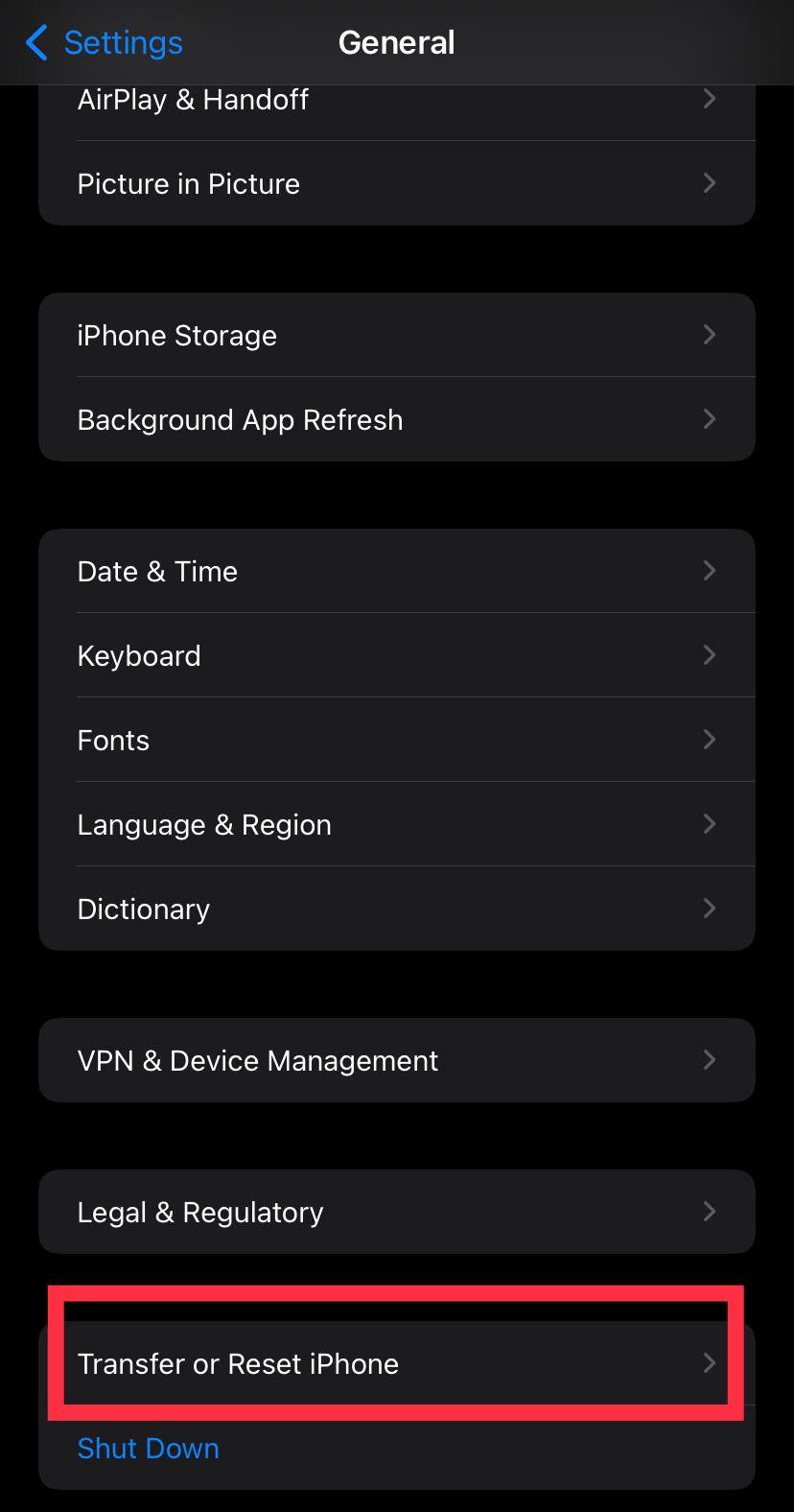In the image, the iPhone settings screen is displayed in dark mode, characterized by a black background with white text. The settings screen currently shows the "General" options, which include: AirDrop, Handoff, Picture in Picture, iPhone Storage, Background App Refresh, Date & Time, Keyboard, Fonts, Language & Region, Dictionary, VPN & Device Management, Legal & Regulatory, Transfer or Reset iPhone, and Shutdown. 

The "Transfer or Reset iPhone" option is emphasized with a highlighted box around it, indicating a potential focus for guidance, possibly by a tech support professional. At the bottom, the "Shutdown" button is displayed in blue text, standing out from the rest of the white-font options, and simply indicating the option to turn off the device. In the top left corner, a back button is visible, offering the option to return to the broader settings menu. The detailed layout and emphasis on specific options suggest careful navigation and perhaps preparatory steps for resetting or transferring iPhone data.